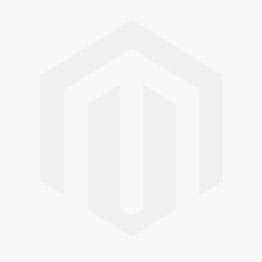The image depicts a digitally rendered interior of a vibrant arcade. The upper part of the scene showcases a ceiling adorned with red neon lights and tiled textures. Dominating the scene is a striking pink neon sign that reads "arcade," casting a colorful glow over three retro-style arcade machines. These arcade systems are lined up against a deep purple wall, each machine distinctly marked by different color bars at the top: purple on the left, red in the center, and blue on the right. The machines' screens are on, displaying blurry, nondescript images, and are equipped with joysticks, button pads, and coin slots on their black bases. To the left of these machines is a large, potted plant with expansive dark green leaves, adding a natural touch to the otherwise electric ambiance. The floor is a light purple, with reflections suggesting a glossy surface. This meticulous blend of neon lighting and vivid colors creates an immersive, nostalgic arcade atmosphere.